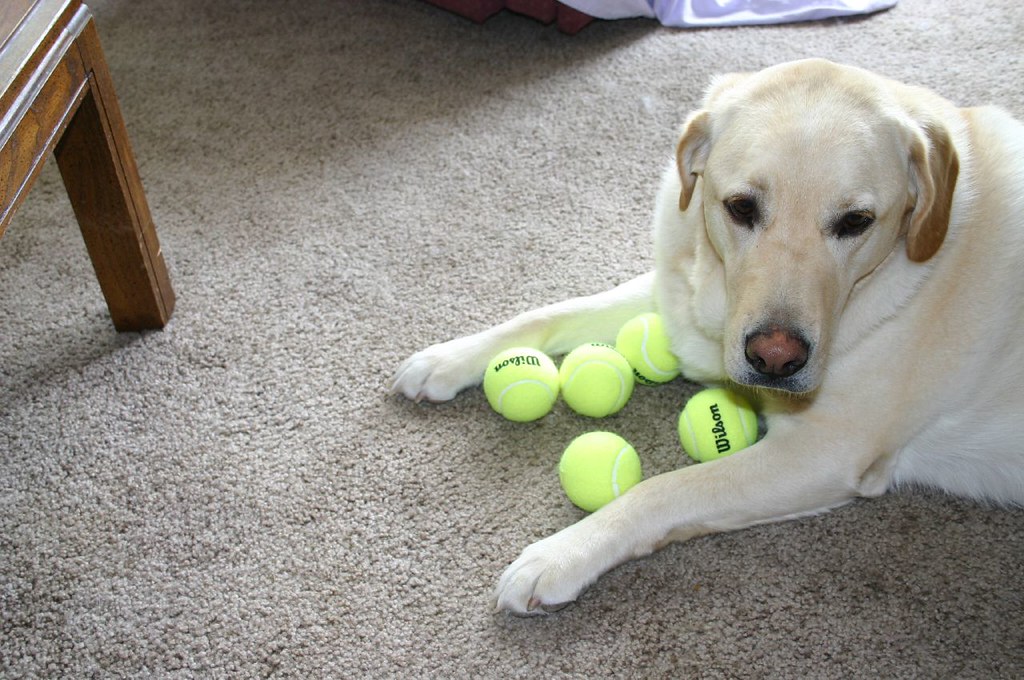In this detailed photograph, we see the front half of a large golden Labrador Retriever, lying down on a light beige carpet. The dog, which has a predominantly white coat with hints of brown fur, especially around its ears, and a pinkish-brown nose, is gazing directly into the camera with its dark, expressive eyes. Framed between its outstretched front paws are five brand new, bright yellow Wilson tennis balls, striking against the neutral carpet. The dog's ears are floppy and slightly browner than the rest of its fur, giving it a distinguished look. At the far left of the image, the wooden leg of either a chair or table is visible, grounding the setting in a cozy indoor space. Toward the top of the photograph, a glimpse of white fabric can be seen, partially cut off but adding to the domestic ambiance. The focus on the dog, with its alert yet gentle demeanor, creates a charming scene of a beloved pet contentedly hoarding its toys.